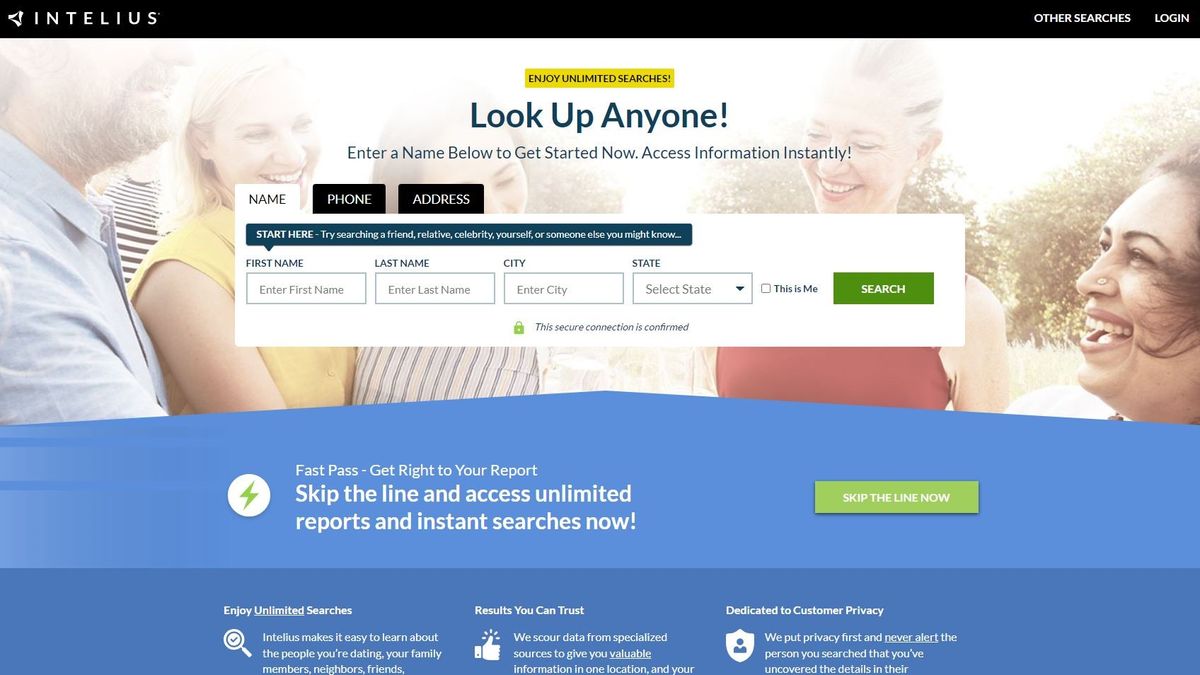**Detailed Caption: Screenshot of Intellius Homepage**

The screenshot captures the Intellius webpage in detail. In the top left corner, the Intellius logo and the name "Intellius" are prominently displayed. Opposite this, in the top right corner, are links to "Other Searches" and "Log In."

Below these, centered on the page, the text "Enjoy Unlimited Searches" is visible. The largest and boldest text on the page is the header "Look Up Anyone." Directly below, the text instructs users to "Enter a name below to get started now. Access information instantly."

A search box is located beneath this instruction. The box has three tabs at the top: "Name" (highlighted against a white background), "Phone," and "Address" (both against a black background). Below the tabs, a smaller box labeled "Start Here" provides search suggestions such as trying to find a "friend, relative, celebrity, yourself, or someone else you might know."

The search form includes text boxes for "First Name," "Last Name," "City," and "State," accompanied by a checkbox labeled "This Is Me." A "Search" button is also present. This entire search section overlays a background photo of five people standing outdoors in a semi-circle, all smiling.

Further down, on a blue background, the promotional text "Fast Pass" is displayed, offering users the option to "Get right to your report. Skip the line and access Unlimited Reports and Instant Searches Now." Adjacent to this text is a button labeled "Skip the Line Now."

The webpage continues with a section reinforcing the benefits of Intellius. The text "Enjoy Unlimited Searches" is reiterated, followed by a description that emphasizes the ease of learning about "the people you are dating, your family members, neighbors, [and] friends." Intellius claims to provide "Results you can trust" by scouring data from specialized sources to offer valuable information in one consolidated location. The final statement underscores the company's commitment to customer privacy: "Dedicated to customer privacy. We put privacy first and never alert the person you search that you've uncovered the details."